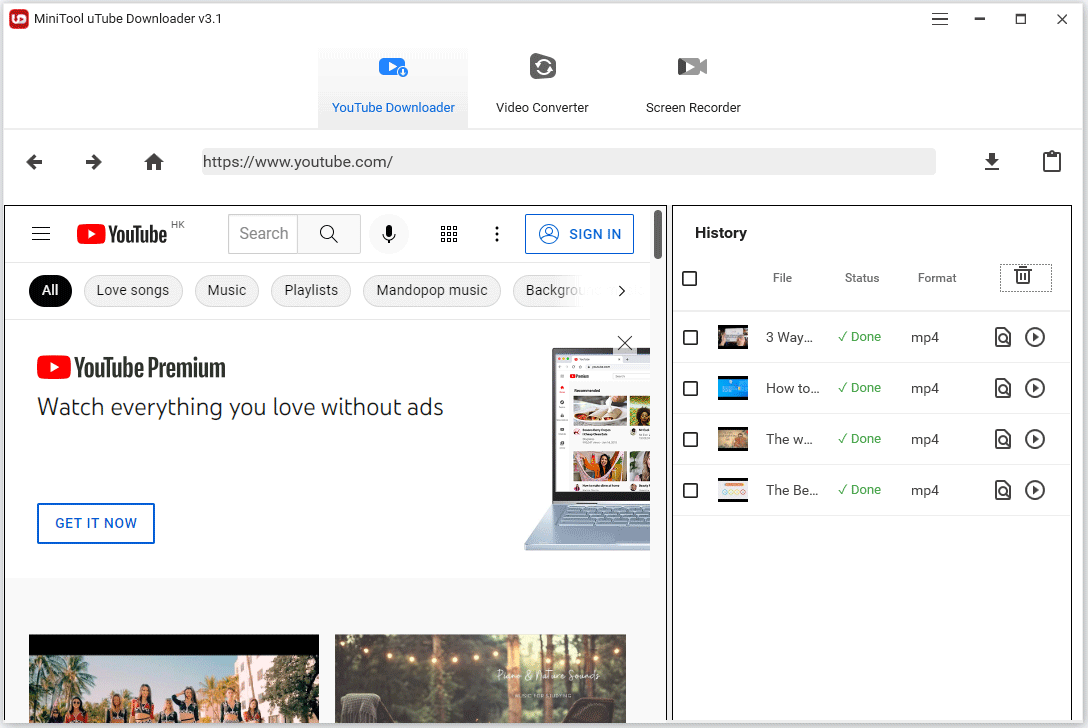The web page presented features a predominantly white background. On the left side, there's a striking red square displaying a white, rotated numeral that resembles either a '6' or a '9'. Adjacent to this square, in bold black text, is the title "YouTube Downloader v3.1".

At the top, the header section includes a grey tab featuring a dark blue YouTube icon with a white, right-facing triangle, and an identification icon in dark blue with an eye symbol. Below these icons, the title "YouTube Downloader" is prominently displayed in blue text.

The interface is divided into two additional grey sections. The first section showcases a white refresh symbol inside a square with the label "Video Converter" below it. Next to it is an icon of a video camera, partly black on the left and grey elsewhere, with another white, right-facing triangle and the label "Screen Recorder".

The central part of the page features a large white area, flanked by black navigation arrows pointing left and right. Below, there’s a home symbol and a grey rectangular input box containing the text "https://www.youtube.com/" in black. This section also includes a download area marked by a black line and a clipboard icon.

On the right, a rectangular section denotes “YouTube HK” or Hong Kong, accompanied by lines indicating settings, a search bar, a microphone icon, and a sign-in rectangle outlined in blue, containing blue text with a silhouette of a person.

Further down the right side, there's a series of oval buttons; the first being black with white text reading "All selected" while others are grey with darker grey text, labeled "Love Songs," "Music," "Playlist," "Mandopop," and "Background" (which is partially obscured), with a right arrow following these buttons.

The web page also promotes YouTube Premium with a red, rounded square symbol containing a sideways white triangle. The text "YouTube Premium" is bold, and beneath it, smaller, non-bold text reads "watch everything you love without ads." A mockup image of a laptop displaying YouTube videos with a silver keyboard is situated below, alongside a blue-bordered button with blue text that says "Get it now."

On the far right, another rectangle has "History" boldly written at the top, followed by a listing with headers "file," "status," and "format." Below these headers, several dotted squares encapsulate black trash can icons, featuring four cascading smaller squares. Next to "file," entries "three way," "how to," "the w," and "the b" are listed. Each entry shows a status marked "done" in green with a corresponding green check mark and lists the format as "mp4." Accompanying each file is an icon of a paper with a magnifying glass and a play button symbolized by a black triangle within a circle and a black border.